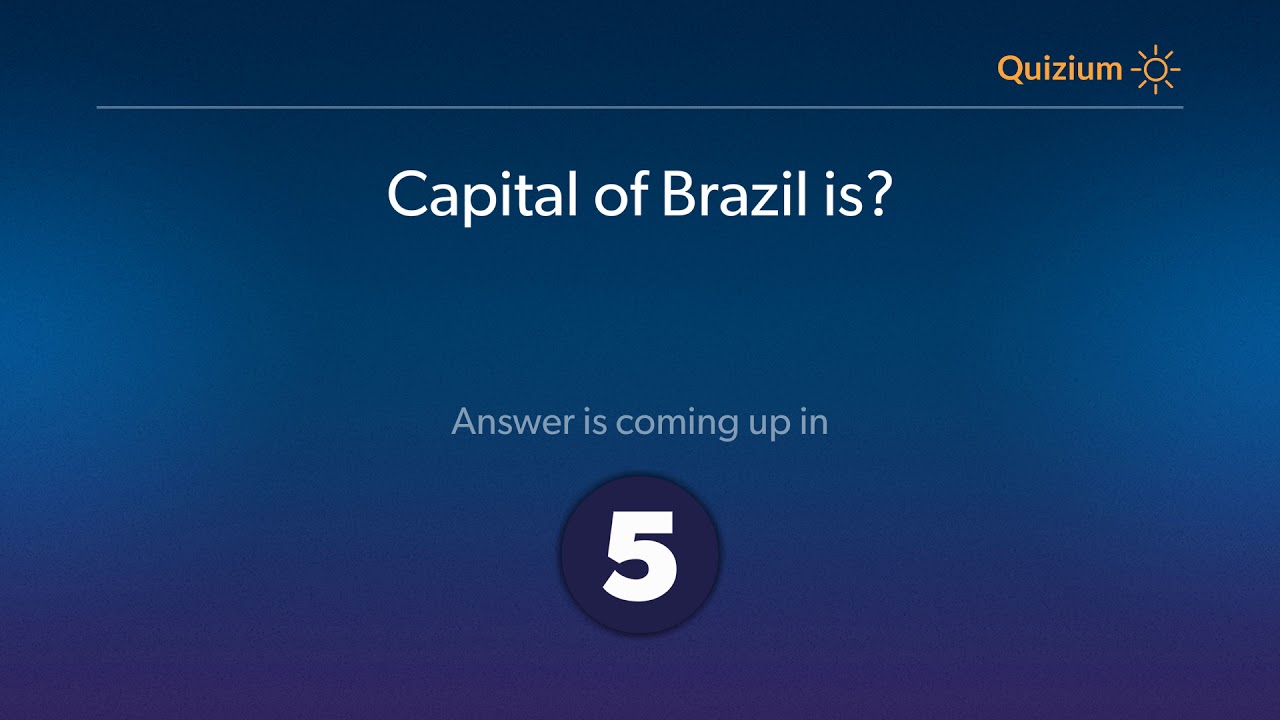The image showcases a webpage interface of a game titled "Quizium," prominently displayed in yellow text on the right side of the screen. The design features a minimalist sun graphic, composed of a simple circle with radiating sunbursts. The game background transitions from dark blue at the top to light blue, with a light blue horizontal line dividing the screen. At the top of the screen, in white text, a trivia question is displayed: "Capital of Brazil is ?" Directly underneath, in smaller light blue font, the phrase "Answer is coming up in:" is clearly visible. A dark blue circular timer prominently displays the number five in white, indicating a countdown. The overall design and elements confirm that the webpage is indeed hosting a trivia game.